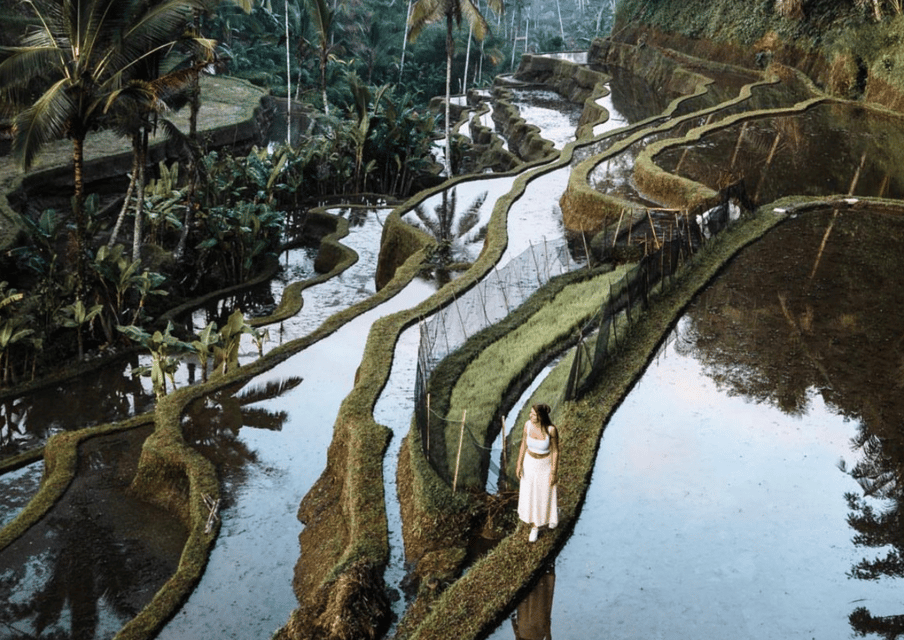This aerial photograph depicts an enchanting, exotic location featuring terraced rice paddies that cascade down towards an open body of water, their flooded levels gleaming brightly under the daytime sun. The landscape is segmented into various twisting and bending strips, resembling pathways that draw the eye towards a lush mountainous grassy range to the right. To the left, a roadway flanked by vibrant foliage leads into the scene, adding a sense of depth and approachability. Nestled within this tapestry of greenery and water is a woman, who serves as the focal point. She wears a long white dress with a brown belt, and her flowing brown hair catches the light as she walks along one of the terraced paths. Palm trees dot the lower levels, contributing to the overall verdant and tropical atmosphere. Protective netting stretched along stakes is visible in some sections, enhancing the intricate agricultural layout. This visually striking image, with its enhanced and poignant colors, resembles a photograph one might find in a high-end travel magazine, enticing potential visitors with its vivid portrayal of serene beauty and lush, cultivated landscapes.